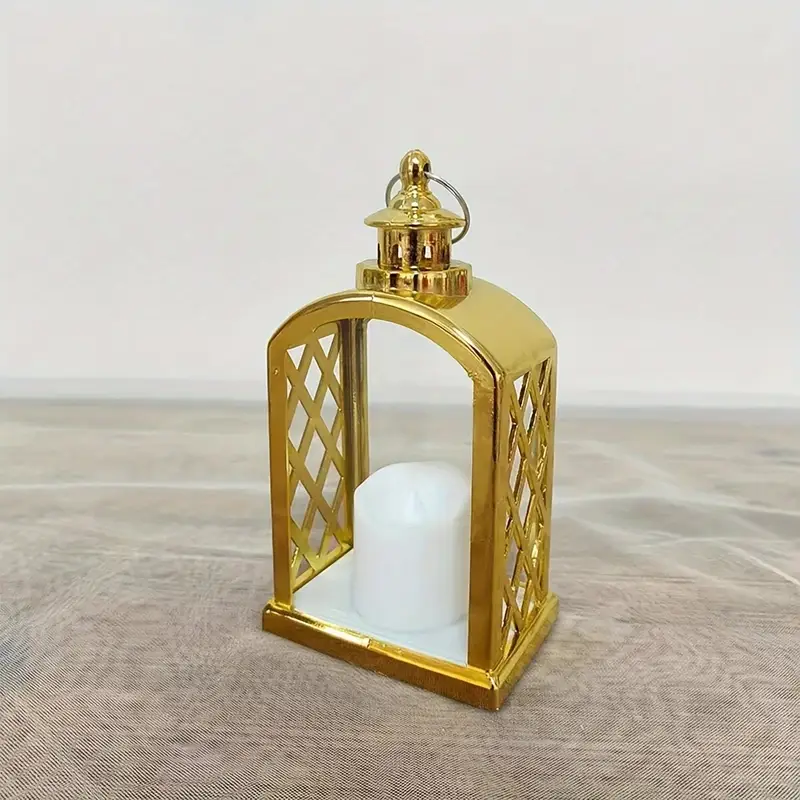A professionally taken photograph features a gold-colored metal candle holder, resembling a small lantern or cage, with a distinctive shape similar to a headstone. The holder has a crisscross diamond pattern on the sides while the front and back are open, revealing a white plastic imitation candle inside. The candle holder has an arch at the top and is topped with a knob and a silver loop for hanging. It rests on what appears to be a gray mesh-like rug or possibly a hardwood surface. There is a white piece of cardboard at the bottom of the candle holder. The background is a plain white wall, enhancing the simple and elegant composition of the scene. No text is present in the image, emphasizing the focus on the candle holder's design and placement.